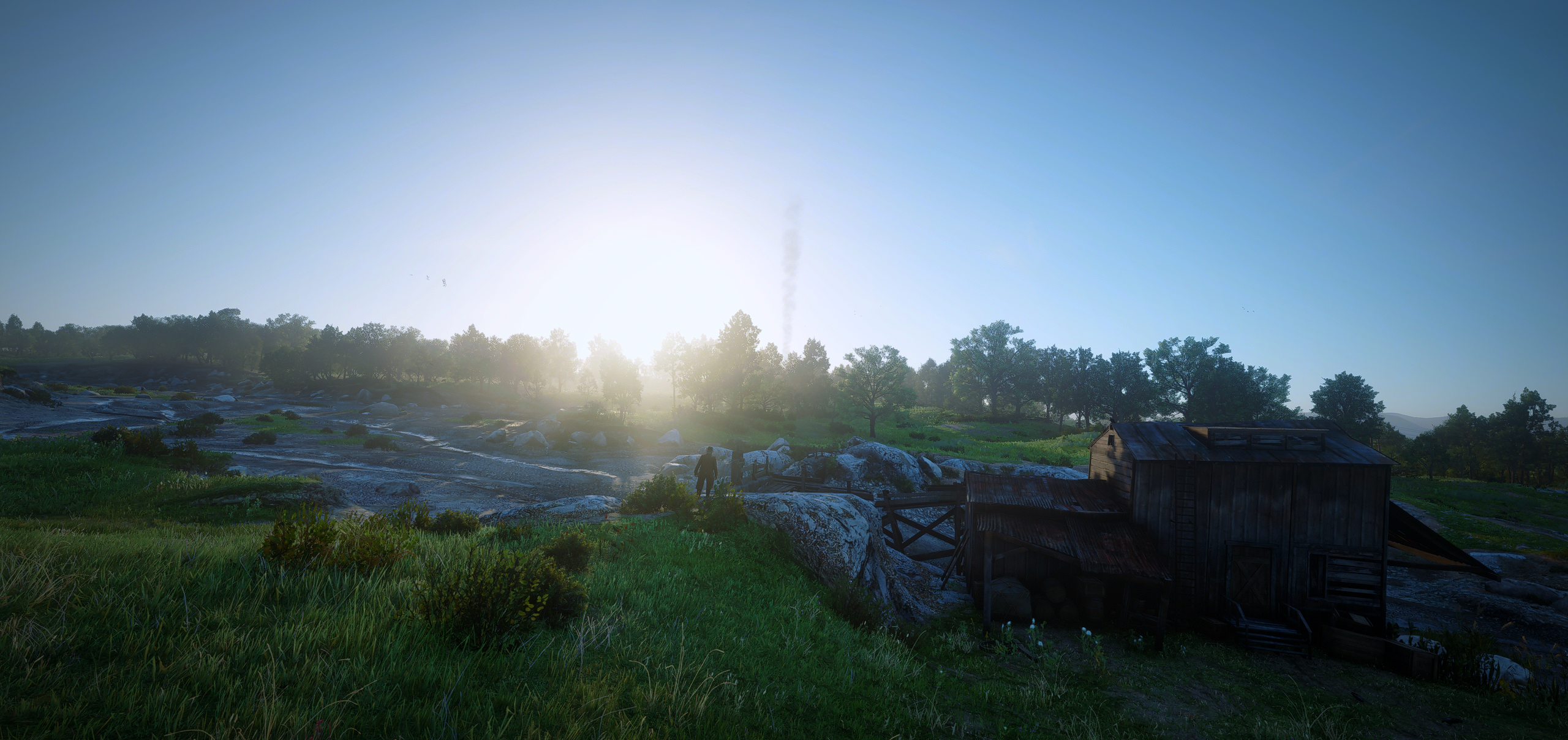This image appears to depict a serene landscape, likely modeled from a video game such as Red Dead Redemption 2, characterized by its remarkable realism and detailed rendering. The scene features vast rolling green hills with trees, both in the foreground and stretching into the background. These hills border a narrow river or stream, with clearly visible low water levels hinting at a previously higher flow. To the right, there's a rustic wooden structure resembling a barn or cabin. The image seems to capture the moment of sunrise, with the sky sporting a vivid blue hue and bright sunlight illuminating the center of the picture. In the distance, beyond the treeline across the river, a plume of smoke rises, possibly indicating a fire or distant camp. Near the river on a rock, a small figure of a man is visible from behind, emphasizing the expansive and open-world nature of the environment. This picturesque scene, with its lush green grass, extensive treelines, and peaceful ambiance, immerses the viewer in a tranquil yet dynamic setting reflective of early 20th-century rural landscapes.